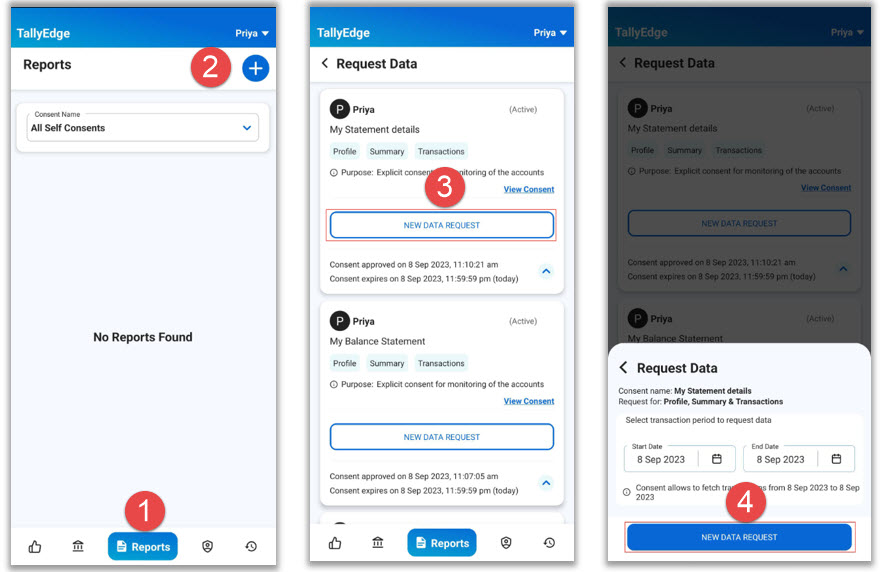This detailed caption describes a mockup of various smartphone screenshots featuring the Tally Edge interface and its functionalities:

---

The image showcases the Tally Edge application interface through multiple smartphone screenshots. At the top, "Tally Edge" is prominently displayed in bold blue letters. To the top-right, the user’s name, "PRIYA," is shown with a drop-down menu beside it in white.

On the left side, a black rectangle houses the word "Reports" in bold black, situated within a white rectangle. Next to it, on the right, there's a large red notification circle with a white numeral '2'. Adjacent to this, another circle in dark blue contains a white plus symbol.

Directly below, a grey rectangle displays "Consent Name". Another rectangle below features a drop-down, marked by a blue arrow, containing the text "All Self Constants" in bold black. A mixture of white and grey rectangles follows, with the text "No Reports Found" in black. This area includes white icons underneath: a thumbs-up, a building, and an orange circle with a numeral '1' in white. Below this, a dark blue rectangle bears the word "Reports". Icons resembling a shield with a silhouette and an eye complete this section.

The subsequent screenshot labeled "Request Data" mirrors the top bezel, which includes a black circle with the text "P-I-Y-A" and "My Statement Details" beside it. To the right, "Active" is mentioned in grey and parentheses. Below the name, three tabs are displayed: "Profile", "Summary", and "Transactions", each tab in light blue with black text. The following section features a grey circle with an eye icon, and black text that reads "Purpose", "Exploit,", and then "Monitoring of Accounts", obscured by an orange circle with a white numeral '3'. A selectable white rectangle with a blue border and text "New Data Request" is highlighted with a red border.

Further down the interface, it states in grey "Consent Approved on 8th SEP 2023, 11:10:21 AM" with the current expiration date "8th SEP 2023, 11:59:59 PM" in parentheses. An up arrow within a light blue background square follows. The user's response follows a similar format, ending with a link "View Consent" in highlighted dark blue with an underline. A rounded dark blue rectangle beneath features white text in all caps: "NEW DATA REQUEST". Additionally, "Consent Approval on 8th September 2023, 11:07:05 AM" and the expiry details are repeated. The right side of this area is greyed out, leading to a popup.

The popup is denoted by an orange circle with a white numeral '4', indicating the fourth step. It begins with the bold black text "Request Data" followed by a left-facing bold black arrow. Next, "Consent Name" in grey is followed by the text "...my statement details" in bold black. New lines follow: "Request From" in grey, bold black "Profile, Summary, and Transactions", and "Select Transaction Period to Request Data".

The left side contains a rectangle labeled "Start Date", displaying "8th September 2023" and a calendar icon separated by a small grey line. Similarly, "End Date" and "8th September 2023" are shown with a calendar icon. The text below mentions consent conditions, partially obscured by the orange circle.

Finally, a dark blue rounded rectangle with all caps white text "NEW DATA REQUEST" is highlighted by a red border, reiterating the fourth step selection.

Overall, the image effectively illustrates the interactive elements and data consent process within the Tally Edge application interface.

---

This caption preserves the detailed description while organizing the information for clarity and comprehensiveness.